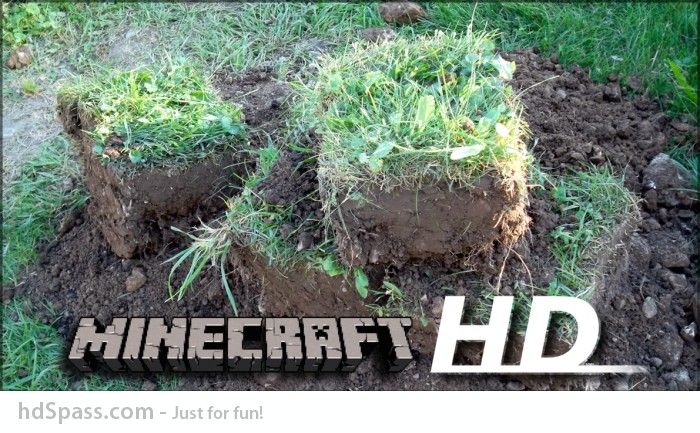This photograph features a patch of ground with visible soil, dirt, and grass. Several chunks of the grassy area have been meticulously dug up and shaped into precise cubes or squares, reminiscent of the blocky terrain seen in the popular video game, Minecraft. Overlaying the image is graphic text; in brown, the word "Minecraft" is written using the iconic Minecraft font style. Below it, the text "HD" appears in white, suggesting high-definition quality. In the bottom corner, a watermark reads "HDspas.com," adding a playful element to the image.